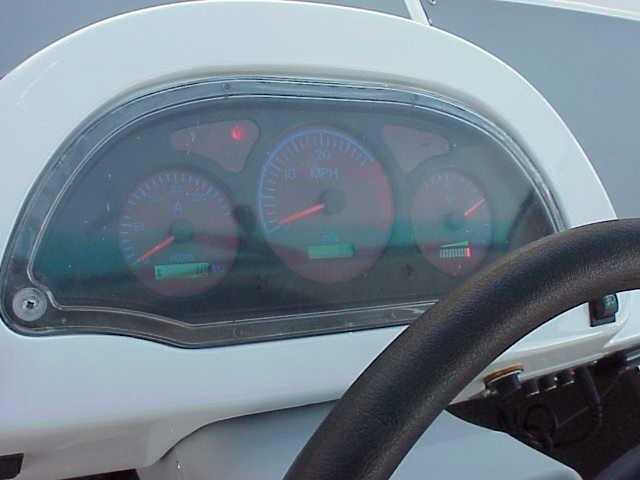The interior of a compact motor vehicle is depicted in this image, focusing on its pristine white dashboard, which appears to be crafted from a plastic-like material. Dominating the dashboard are three major circular gauges, all encased behind a clear, plexiglass-like cover. The largest gauge commands the center position with its prominent size and features. This central gauge is marked with a blue line, and has blue indicator lines highlighting the numbers 40 and 70, signifying speeds in miles per hour (MPH). A red hand is poised to measure the vehicle's speed, though it currently rests at zero. Additionally, there is an unused display bar present within this gauge.

To the left, another similar gauge is adorned with various lines and a red hand, but its specific function remains ambiguous. Notably, it includes the letter 'A'.

The gauge on the right side is partly obscured, rendering some details unreadable. However, it displays a line that ascends from lower to upper ranges. At the top of this gauge are two arrow-like indicators, one of which is illuminated by a red light.

The intricately designed dashboard, with its combination of functional dials and highlighted indicators, suggests a well-equipped and technologically informed vehicle space.